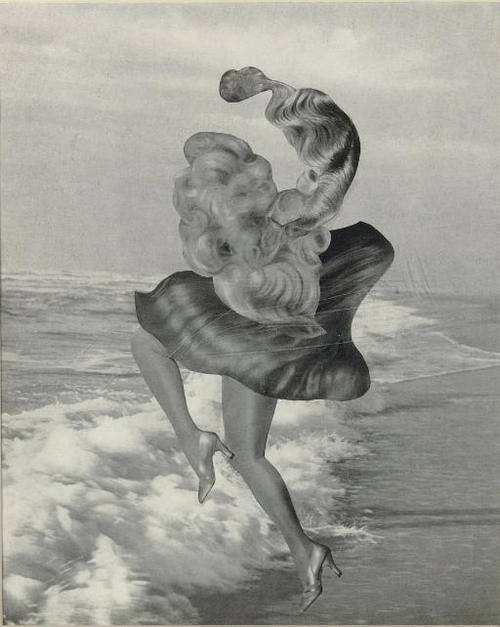This captivating black and white artwork presents a surreal scene that blurs the line between photography and drawing. Set against a backdrop that looks like a photograph of the ocean, complete with dark gray waves washing onto the shore and a cloudy sky in various shades of gray, the central focus is a woman in a dynamic pose. She is viewed from the back, seemingly suspended in the air with her left leg lifted and poised on the tip of her right toe, clad in high heels. Her skirt and hair appear distorted and windswept, merging into abstract, twisted shapes that obscure her upper body and face. The skirt is a chaotic swirl, resembling a cloth caught in a strong gust of wind, while her hair extends and mingles with the distortion, creating a tangled, fluid mess. The detailed depiction of her legs stands in stark contrast to the amorphous blend of her dress and hair, making this piece a uniquely imaginative fusion of realism and surrealism.